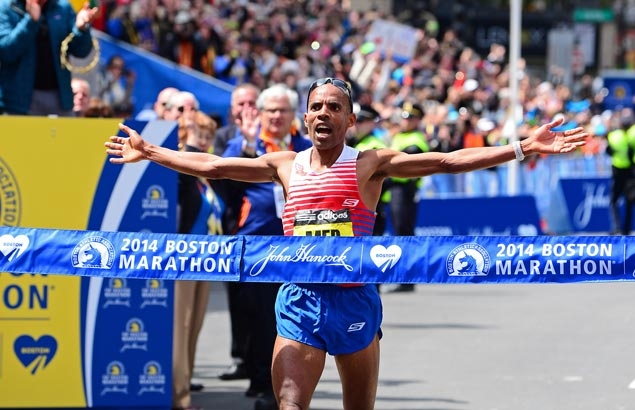The image captures the exhilarating moment a black male runner, a participant in the 2014 Boston Marathon, sprints towards the blue finish line ribbon adorned with "2014 Boston Marathon" and "John Hancock" in white text. He is clad in a red and white running top and blue shorts, with sunglasses perched on his bald head. With his arms wide open and a look of triumph on his face, he is seconds away from breaking the tape with his chest. Spectators in the background, blurred out and seated in blue bleachers, cheer him on fervently, waving their hands and holding signs in celebration. Additional onlookers, including individuals with distinctive white and red hair, stand nearby, their expressions captured in clear focus as they witness the runner's monumental achievement.